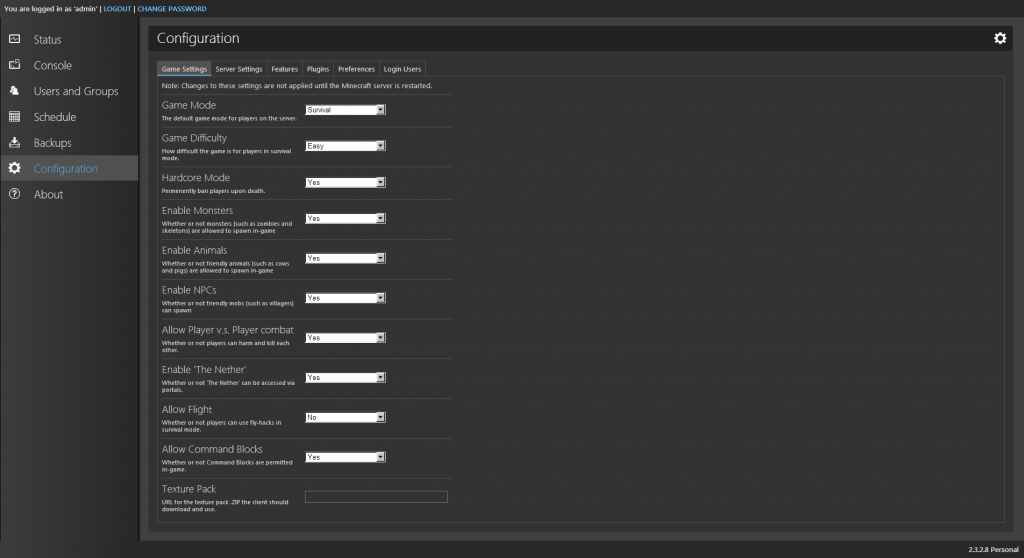This image is a screen capture of a computer application, likely displayed on a tablet, desktop, or laptop due to its landscape orientation. The screen features a dark gray background with slightly darker gray accents in the left-side vertical menu and in thin strips along the top and bottom edges.

The left-side menu presents several options: "Status," "Console," "Users and Groups," "Schedule," "Backups," "Configuration," and "About." The "Configuration" option is currently highlighted in light blue, indicating it is the active selection. Navigation buttons, also in light blue, are located in the upper left corner of the screen.

The main area of the application, which occupies the majority of the screen, is a slightly lighter medium-tone gray. It showcases a series of configuration settings aligned vertically. Each setting has a header, a brief description, and an associated drop-down menu box on the right. 

Most drop-down boxes are set to "Yes," except for the topmost option, which is unreadable due to its small text, and the penultimate option, which is set to "No." There are ten drop-down menu items in total, followed by an eleventh option featuring a search box where users can type to search for additional settings. The overall color palette of the application is composed of shades of gray, white, and black.